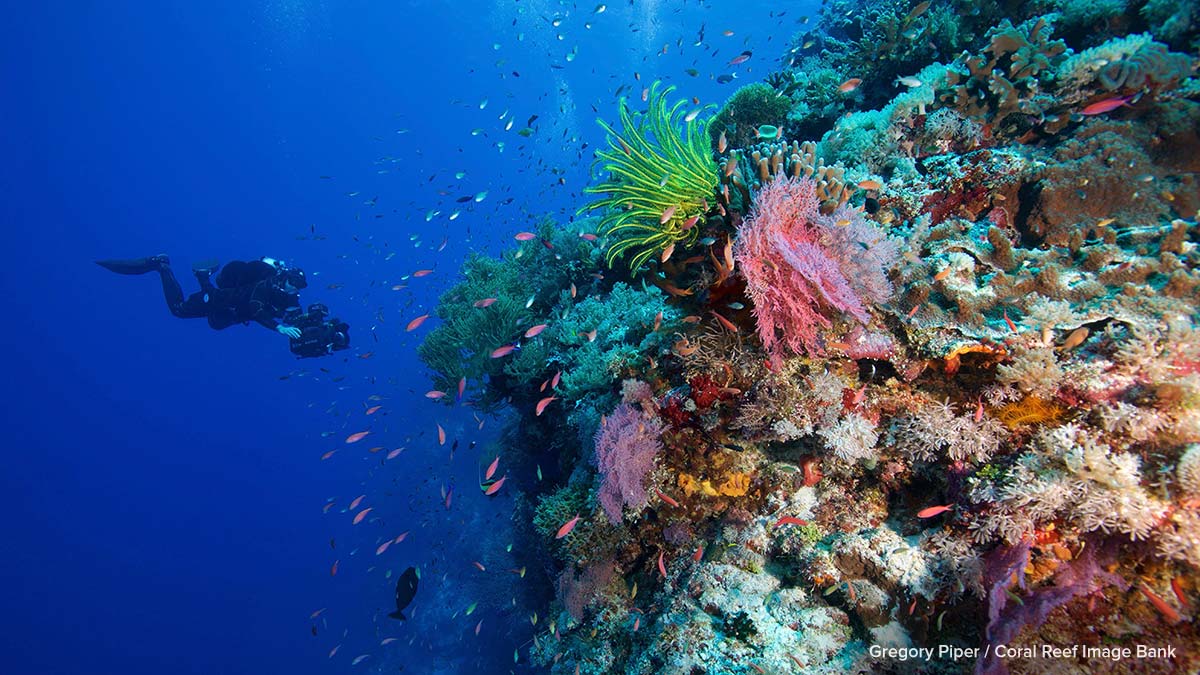This underwater photograph captures a vibrant coral reef set against the deep blue ocean. The reef, located on the right side of the image, bursts with a spectrum of colors including greens, aqua blues, pinks, purples, and whites. It showcases an array of marine life, with several small fish adding to the scene's vibrancy; some fish are strikingly hot pink, while others are more subdued in coloring. On the left side of the image, a fully outfitted scuba diver can be seen maneuvering in the water, seemingly holding a camera to capture the breathtaking underwater landscape. The diver's flippers, tank, and camera gear are clearly visible, suggesting he is documenting the natural beauty around him. At the bottom right corner of the image, text reads "Gregory Piper Coral Reef Image Bank," indicating that this stunning photograph is part of a curated collection. The colors of the coral and fish appear entirely natural, not enhanced by artificial lighting, highlighting the true beauty of this underwater ecosystem.